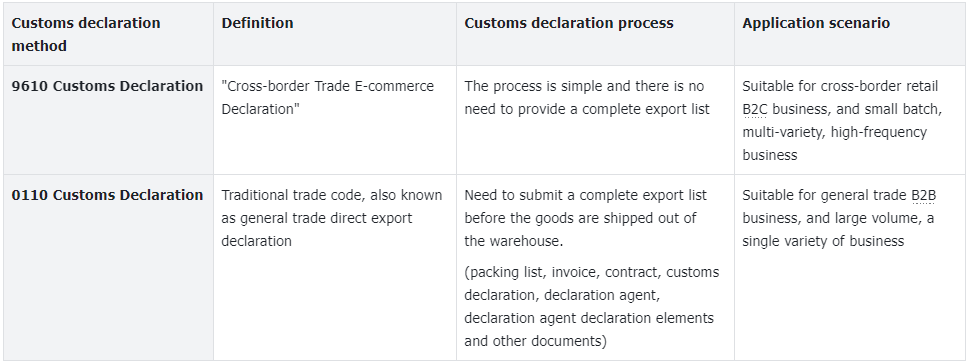The image is a detailed chart depicting different customs declaration methods, their definitions, processes, and application scenarios. The chart is divided into columns titled "Customs Declaration Method Definition," "Customs Declaration Process," and "Application Scenario." The rows are labeled "9610 Customs Declaration" and "0110 Customs Declaration."

In the 9610 Customs Declaration row, it is described as a Cross-Border Trade E-Commerce Declaration, where the process is streamlined and does not require a complete export list. This method is suitable for cross-border retail, B2C business, small batch, multi-variety, and high-frequency operations.

The 0110 Customs Declaration, identified as the Traditional Trade Code or General Code, involves direct export declaration. This method requires the submission of a complete export list before the goods are shipped out of the warehouse. It is suitable for general trade, B2B business, and large volume, varied business types.

The chart’s titles are highlighted with grey backgrounds and bold black letters, while the detailed information in the boxes is presented against white backgrounds.